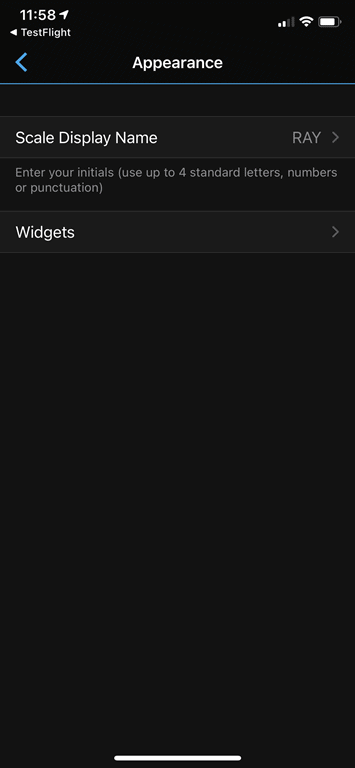The image appears to be a screenshot taken from a smartphone, featuring a predominantly black background. In the top-left corner, the time is displayed as "11:58." Directly beneath the time, the words "TestFlight" are visible. On the top-right corner, there are four signal bars, with two bars filled in and two not, accompanied by a Wi-Fi icon and a battery indicator showing approximately 80% charge and colored white.

Below this header, the title "Appearance" is prominently displayed in white text, with a blue underline. Further down, there is a grey bar containing the words "Scale Display Name" in white text. To the right of this text, the name "Ray" is displayed. Below this section, a prompt reads: "Enter your initials (use up to four standard letters, numbers, or punctuation)."

Further down, another grey bar is present, labeled "Widgets" on the left, with a right-pointing arrow on the far right indicating interactive functionality. 

The bottom portion of the image, approximately 80%, consists of a solid black area, giving a minimalistic appearance. At the very bottom of the screen, a solid white line is centered, possibly indicating a swipe gesture area or a navigation bar.